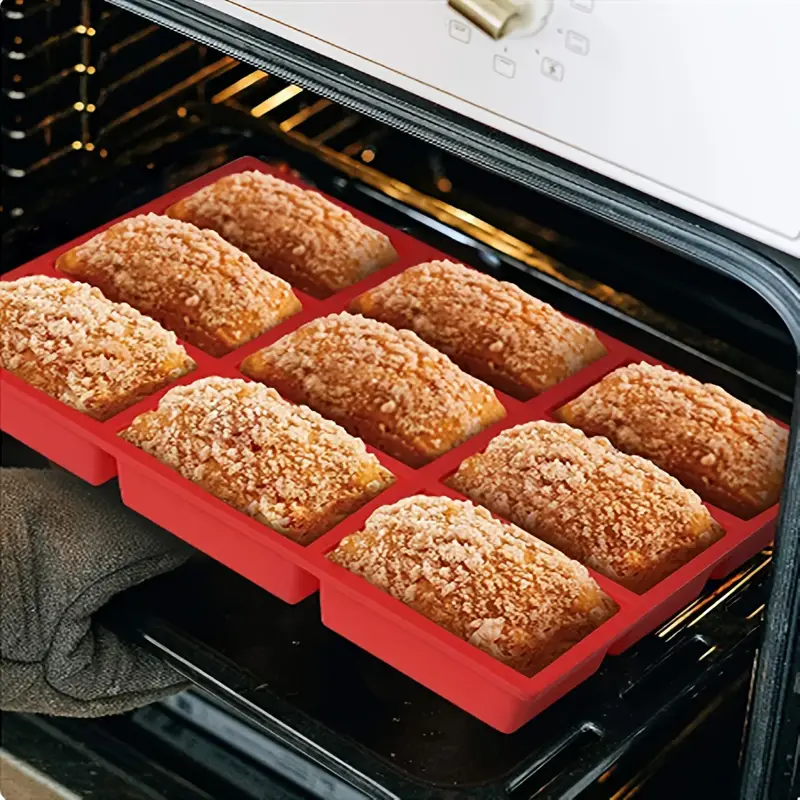This detailed image captures the moment someone is pulling out a bright red mini loaf pan from a black oven with silver racks, using gray oven mitts. Inside the pan, there are nine small, brown-topped loaves of bread or possibly sweet baked goods, such as coffee cakes, given the appearance of streusel-like crumbles on top. The oven light is turned on, casting a warm yellow glow on the scene, which enhances the textures and colors of the baked items, the pan, and the oven interior. The loaves are fluffy and brown, with a slightly crunchy appearance on top, suggesting a delicious, freshly-baked treat.